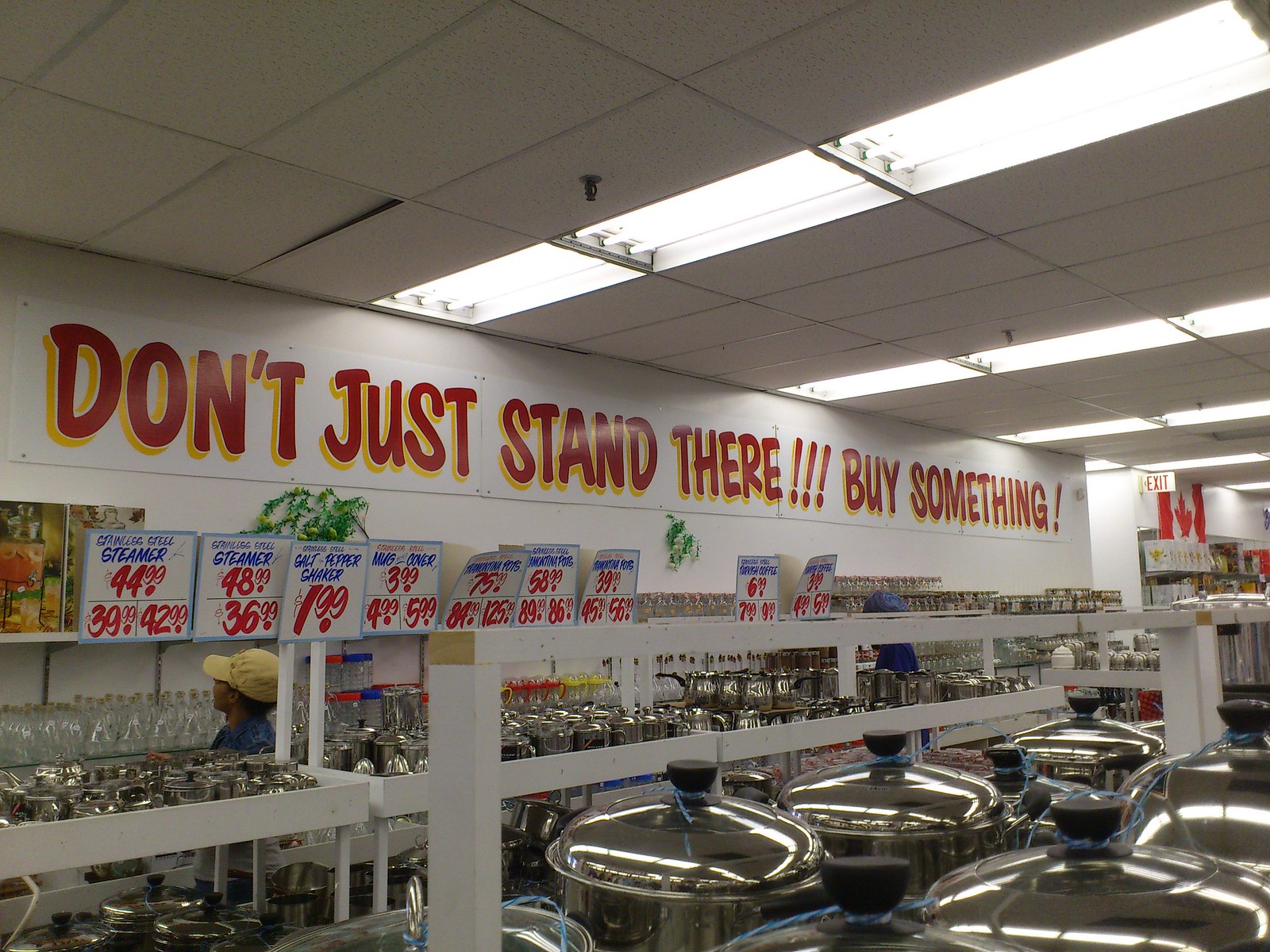The photograph depicts the interior of a retail space with a grey wall. Prominently featured on the wall is a bold, painted message in red print with a yellow outline that reads, "Don't just stand there!!! Buy something!!!" Above this sign, a tiled roof is visible, with one tile appearing slightly loose. Embedded in the ceiling are fluorescent lights, providing illumination to the space.

Below the sign, various plants and greenery add a touch of nature to the scene. Scattered along the wall are several price signs in red and blue, though they are challenging to read from this angle. In the background, grey metallic items, likely cutlery or cookware, are arranged on distant shelves. A closer view in the bottom left corner reveals a collection of metallic round pots with lids. These pots feature small, black round knobs on top, indicative of their utility in a kitchen setting.